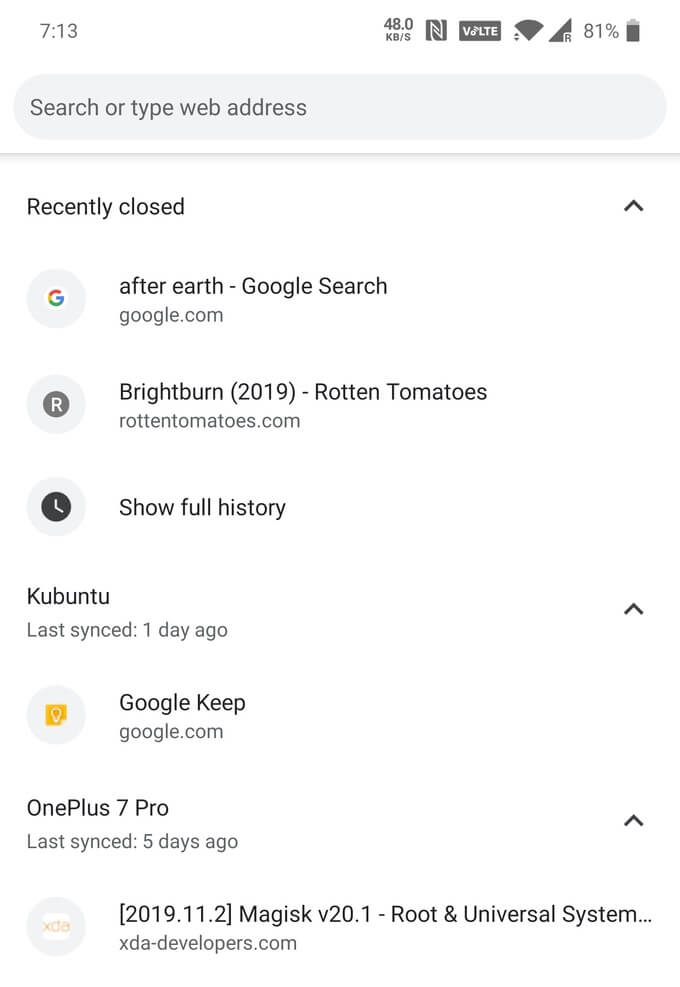The top left corner displays the time, "7:13," in light gray. To the right, there is a bold gray text, "48.0 KB/S," indicating data speed. Adjacent to this, a dark gray square with a Z or N shape containing two lines inside it is visible. Further right, there's a dark gray rectangle marked "VOLTE" in white, with the "O" styled as a speaker icon. Next, a full-signal Wi-Fi icon, full cellular service bars, and an "81%" battery percentage icon, followed by a battery image depicting about 80% charge, can be observed.

Below this, an oval-shaped search bar with a gray background is found. Inside, the dark gray sans-serif text reads "search or type web address." Underneath the search bar, "Recently Closed" is written in black. Toward the left, a gray circular icon with the Google "G" logo is present, subtly outlined in white. To its right, "After Earth - Google search" appears in black text, with "google.com" written in small gray lettering beneath it.